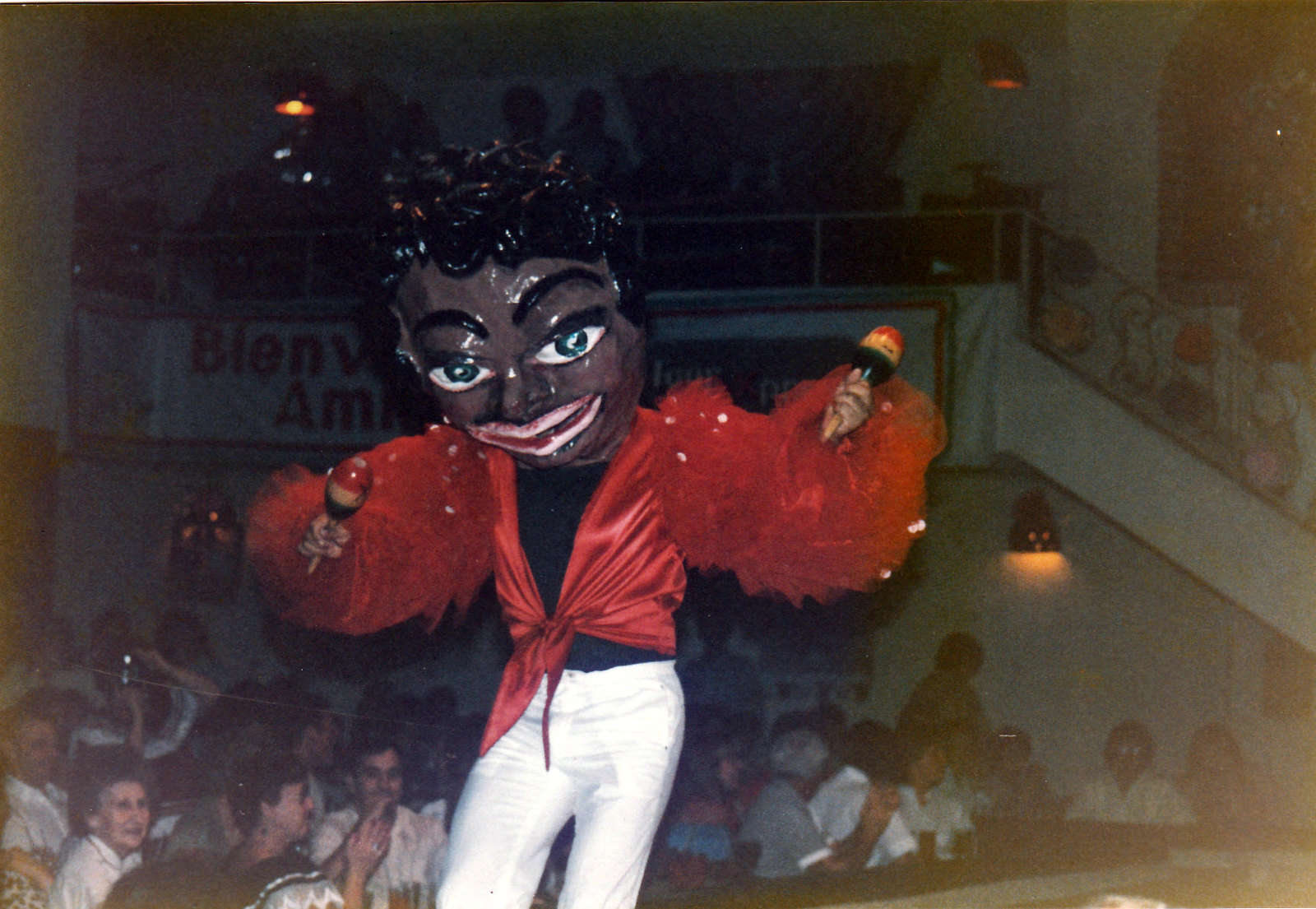In this captivating photograph, a performer, possibly a woman, dazzles on stage, donning a strikingly large mask depicting a black woman with black hair, dark brown skin, and pink lips. The performer is dressed in a black top layered under a red top with extravagant, fluffy ruffle sleeves, and white pants. She energetically shakes rattles, featuring red, yellow, and black stripes, in both hands, reminiscent of maracas. The scene unfolds in what appears to be a dance hall, bar, or lounge, with an attentive audience of men and women seated at tables, engrossed in the lively spectacle before them. The performer evokes a Michael Jackson vibe, suggesting a possible homage or parody, blending vibrant costume elements with dynamic stage presence.